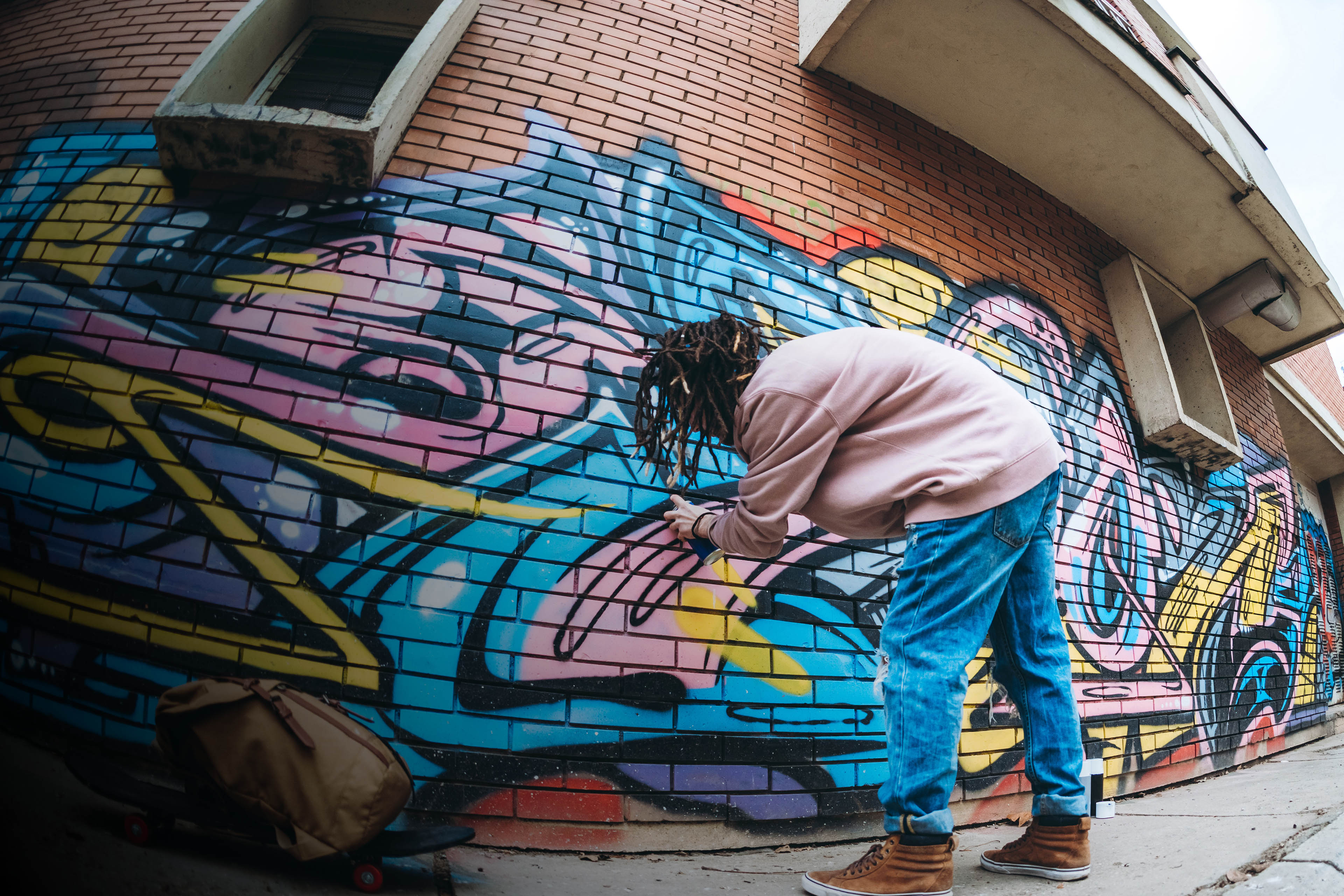In this vibrant daytime photograph taken outdoors, we see an African American street artist with long black dreadlocks actively spray painting on a red brick wall. He is dressed in a light pink hoodie or sweater, blue jeans, and brown sneakers. A brown bag, presumably holding additional spray paint cans, rests on the sidewalk next to him, which has a few visible cracks. The image, captured with a fisheye lens, features a broad view of the building's side, adorned with multiple windows and revealing a snippet of blue sky in the upper right corner. The graffiti, splashed with colors of blue, yellow, pink, and black, includes large abstract lines and swoops, with the only discernible character being a letter "Z." Concrete features protrude from the building, possibly windows or structural elements, adding depth to the scene.